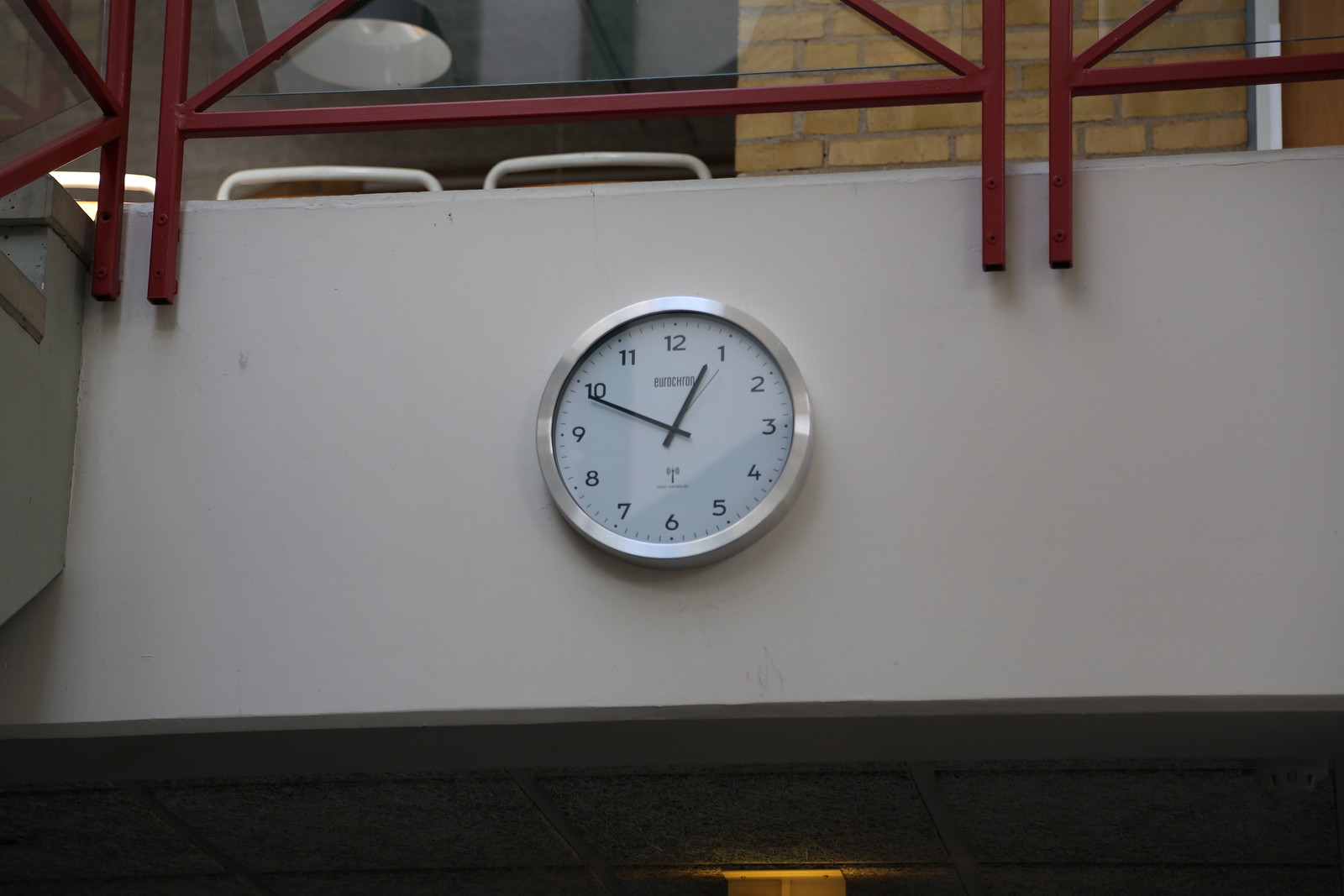The image captures a modern, minimalist clock suspended between two levels of a building. The clock, which appears to be made of stainless steel, features a highly reflective face and is mounted on an off-white, painted cement wall. To the left of the frame, a staircase ascends towards the upper level, flanked by maroon or dark red railings.

The clock face itself is detailed with bold, sans-serif numbers — 12 at the top and 6 at the bottom — and in between these numbers, thicker tick marks denote the hours, while smaller ticks indicate the minutes. The hour and minute hands are black, and although the clock bears a brand name at the top, it's difficult to decipher. Towards the bottom of the clock face, there is a symbol that likely represents a wireless synchronization feature, suggesting that the clock syncs automatically via an atomic clock signal.

The upper portion of the image reveals brown bricks with matching brown mortar, adding a touch of rustic charm to the otherwise contemporary setting. There are metallic, possibly brushed steel, objects that appear to be chair backs or some other fixtures.

In the upper left corner of the image, a lamp is visible with a white bulb encased in a shade that looks dark green or black from the outside. Near the bottom middle of the frame, another light source is partially visible, illuminating the area under the stairwell, which remains mostly in shadow.